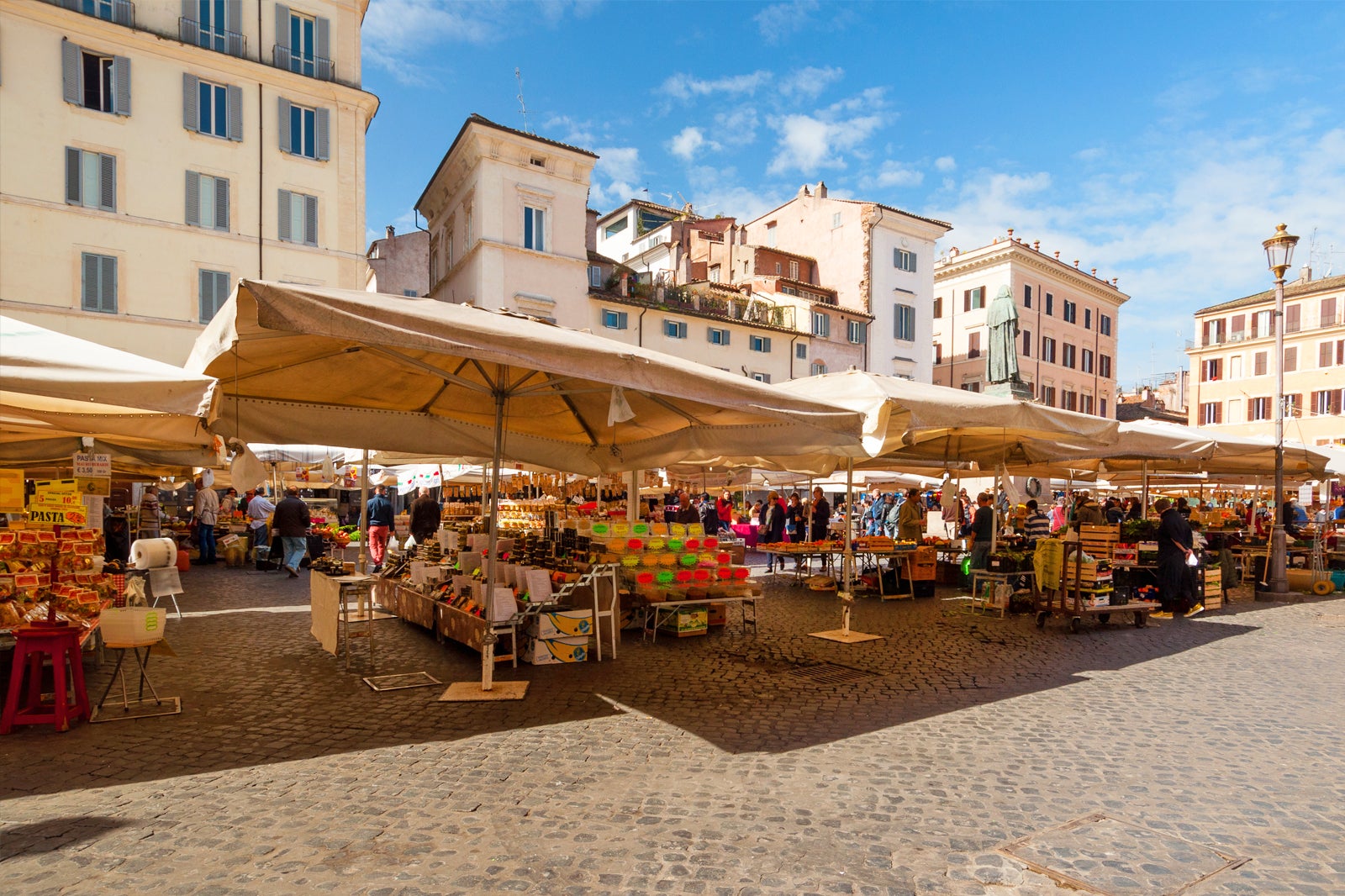The image portrays a bustling outdoor farmer's market set against a backdrop of four to five-story white buildings, possibly apartments, with a blue sky and scattered clouds overhead. The street, paved with stones and cement, hosts several tan-colored canopy tents, resembling large square umbrellas that provide shade to the vendors and shoppers beneath. Under the canopies, rows of diverse food items are displayed, including tables labeled with ‘pasta’ and shelves stacked with colorful containers in red, green, yellow, and orange. There are bags and even a banana box visible among the goods. Shoppers mill about, inspecting the offerings and engaging with sellers. In the background, another row of similar setups extends, adding to the lively atmosphere. A street lamp stands on the right-hand side, partially blending into the scene of people enjoying their market day.